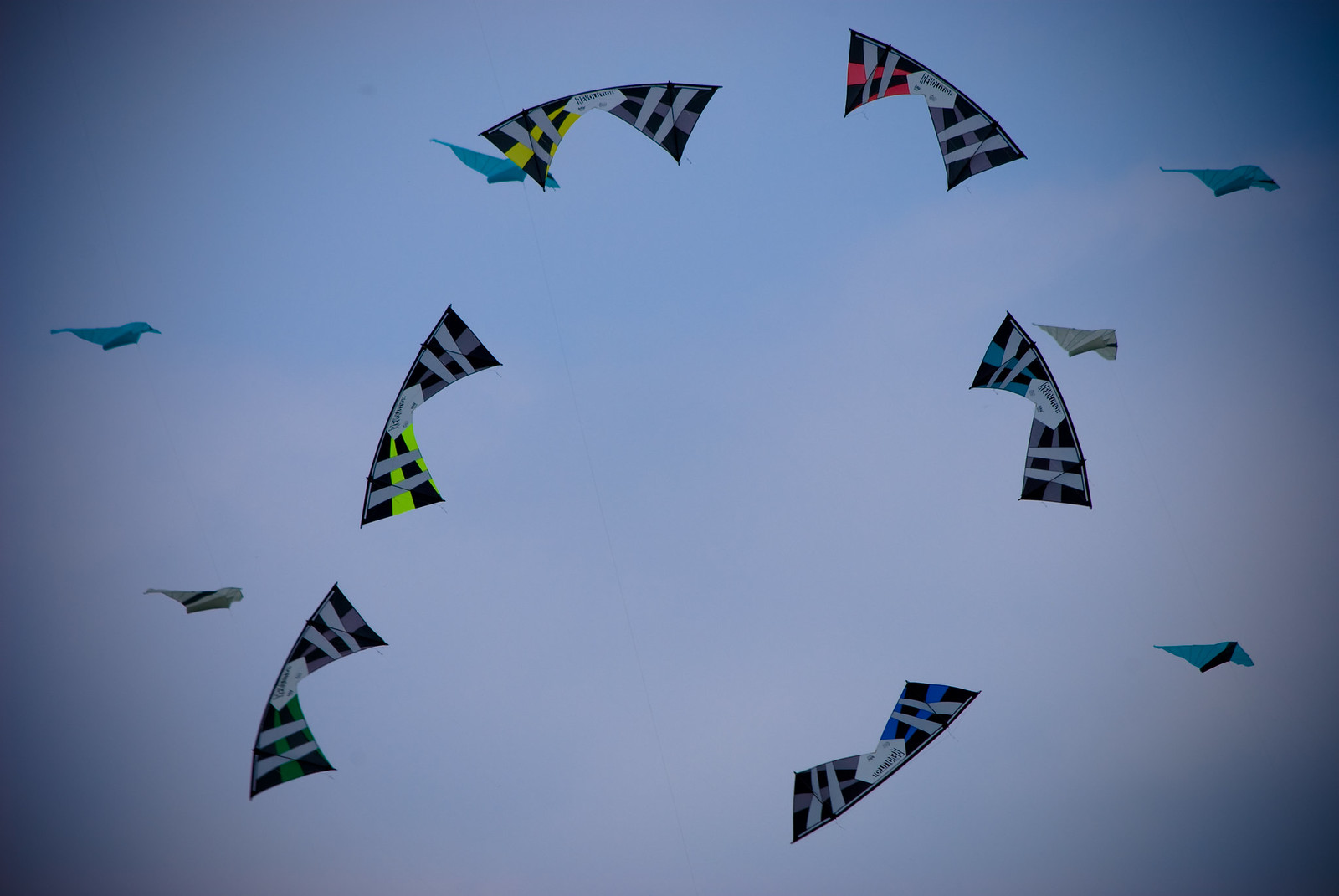This image portrays a group of kites soaring high in a muted, somewhat dull sky. The sky transitions from blue at the top to a cloudy white towards the bottom, and the scene appears to be captured from the perspective of someone standing on the ground, looking up. There are a total of 11 kites visible, with distinct differences in size and design.

In the foreground, six larger kites dominate the middle of the frame, each featuring vivid accent colors against a base of black and white stripes. These kites include one in green, white, and black; two in yellow, black, and white; one in red, black, and white; one in blue, black, and white; and one in purple, black, and white. The design of these kites is unique, resembling a bow-tie shape with a rectangular structure that bends slightly. 

Surrounding these larger kites are five smaller ones. The exact colors of these smaller kites are more challenging to discern, but they are noted to be white, teal, or possibly turquoise. These smaller kites appear to be arranged in a more random pattern around the larger ones, adding to the abstract beauty of the scene.

The backdrop sky provides a muted, almost dusky tone, creating a contrast with the sharply colored kites. The overall ambiance suggests either a late afternoon or early evening setting, enhanced by the dark vignette around the edges of the photo. Despite the lack of visible kite strings, the image convincingly appears to be a natural capture of kites in mid-flight, although some ambiguity remains about whether it might be a photoshopped or AI-generated artwork.